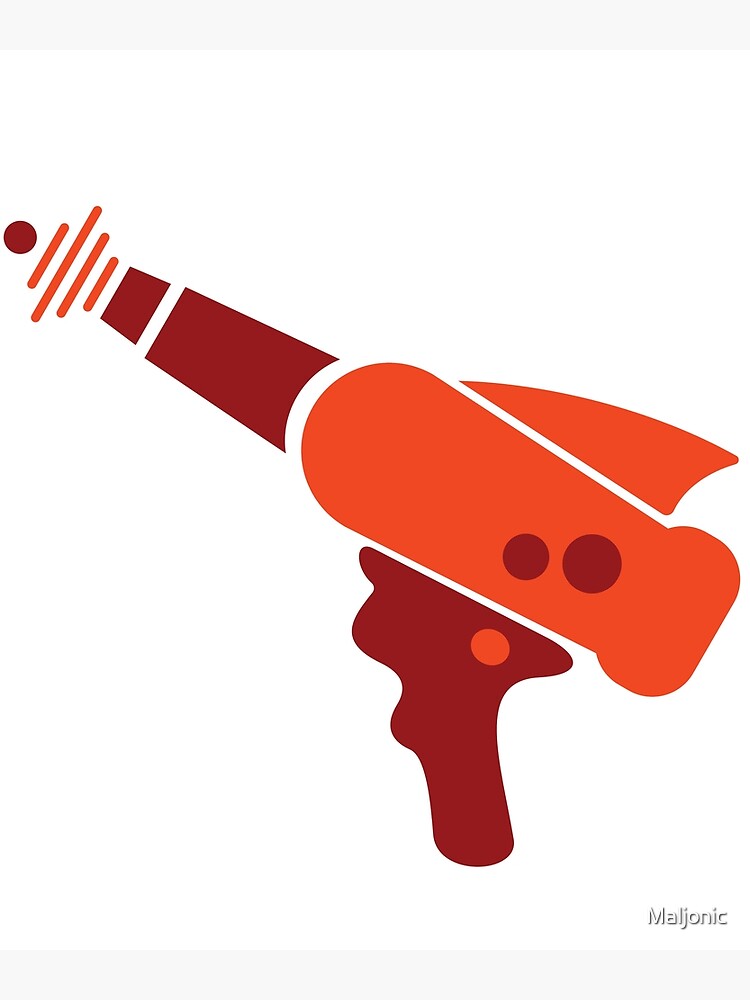The image displays a simple, clip-art style artwork with a white background. Enclosed within a rectangular frame—twice as long on the sides as it is tall— the artwork features thin, light gray banners at both the top and bottom edges. At the bottom right corner, the word "Malgenic" is written in white text with a black outline. The central piece of the image is a red, retrofuturistic laser gun composed of various distinct shapes with white gaps between them, forming a disjointed yet cohesive whole. The grip of the gun is a dark reddish-orange with a light orange circle near the trigger area. The barrel, which is directed toward the top left, is dark orange at the front with an orange circle at the muzzle, from which three light orange diagonal lines suggest laser emission. The back end of the gun resembles a rocket ship with a fin on top, colored in a medium orange, and decorated with two darker orangey-red circles.